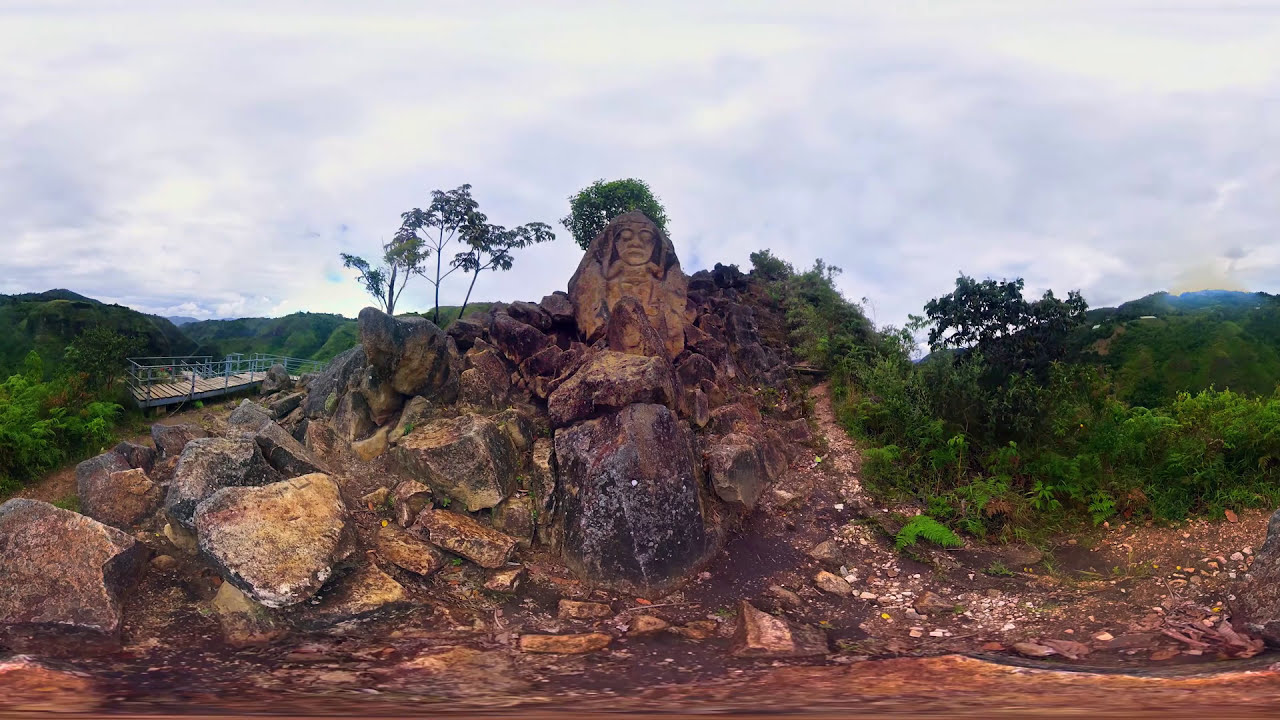The image depicts an ancient, outdoor memorial site set within a lush, forested area. Dominating the center is a large, weathered rock structure featuring an intricately carved figure of a person, likely from an ancient civilization. The figure, with large eyes and a possible crown or flowing hair, stares downward, hands near its head, adding a sense of historical depth.

Surrounding this central rock are numerous jagged and eroded stones, some with distinct etchings, suggesting a once-significant cultural or ceremonial site. In the background, vibrant green trees and various shrubs fill the landscape, hinting at a rainforest or similarly verdant environment. Distant mountain ranges add to the scenic beauty, their greenery visible despite the overcast sky.

To the left of the image, there's a bridge or large platform, guiding viewers’ eyes towards the ancient centerpiece. Above, the sky is predominantly cloudy with patches of blue peeking through, indicating that the photo was taken during the daytime. The rich palette of colors includes various shades of green, gray, tan, brown, and hints of yellow and blue, emphasizing the natural and historical harmony captured in the scene.